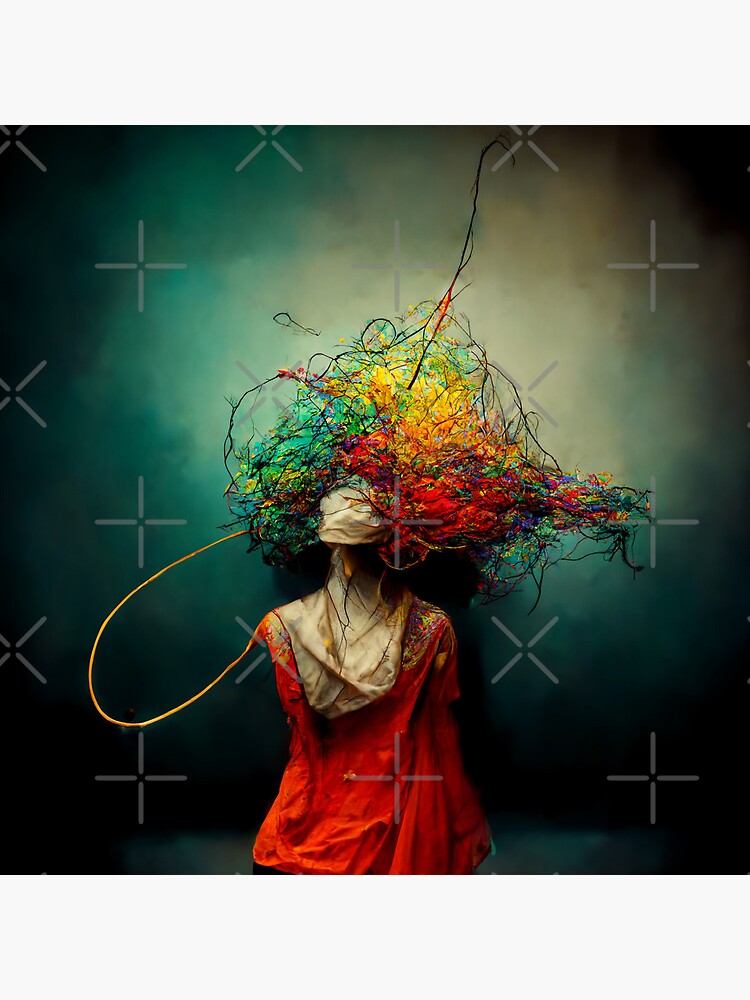The image depicts a mixed-medium piece of art featuring a figure resembling a woman, crafted from various fabrics and materials. The figure is adorned in a vibrant red jacket or dress with intricate floral designs and gold buttons, complemented by a yellowish-ivory colored scarf draped around its neck. Atop the figure’s head is a mismatched hat, extravagantly decorated with an array of ribbons and threads in reds, purples, teals, greens, yellows, and blues, creating a wild and chaotic hair-like arrangement. The background transitions from dark green fading to lighter green or teal, then to beige and black, giving an impression of light projection. Lightly grayed X's and crosses are also faintly visible in the background, adding to the complexity and depth of the scene. The entire composition feels like an artistic blend of sculpture and painting, offering a visually rich and intricate display.